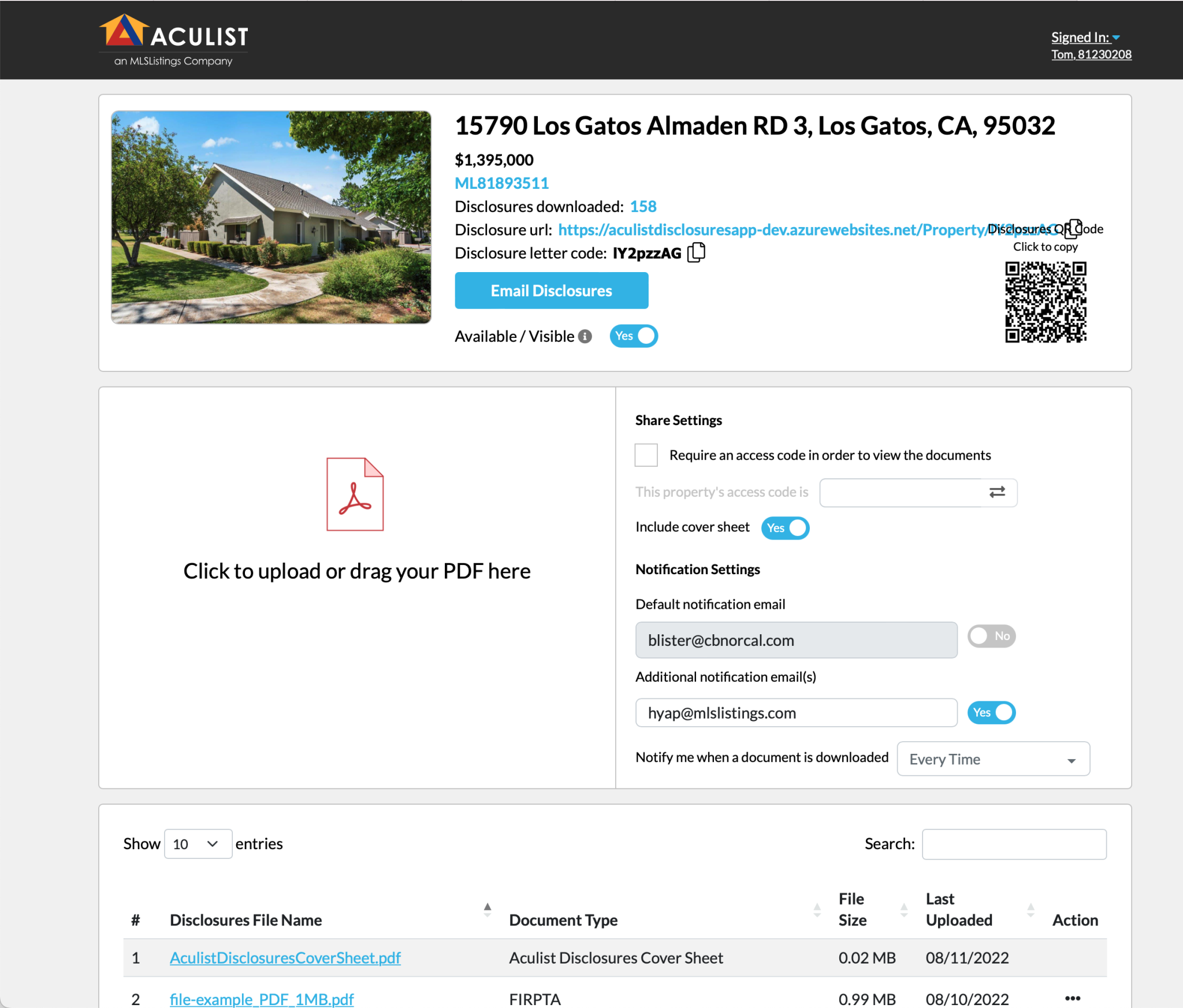AccuList Real Estate Listings Website: Detailed Listing for 15790 Los Gatos, Al Marden Road 3, Los Gatos, California 95032

This page on the AccuList website features an exclusive real estate listing for a house located at 15790 Los Gatos, Al Marden Road 3, Los Gatos, California, 95032. The property is currently listed at a price of $1,395,000. Visitors to this page have the option to download the available disclosures, or alternatively, email the disclosures directly to themselves or interested parties. 

Furthermore, the seller appears to be in the process of creating the listing, having recently uploaded a disclosure cover sheet and a FIRPTA document on November 8, 2022. Additionally, there is a QR code available on the page for easy access to listing details on mobile devices. The page also features various settings for managing the listing efficiently.

< Photo of the property >